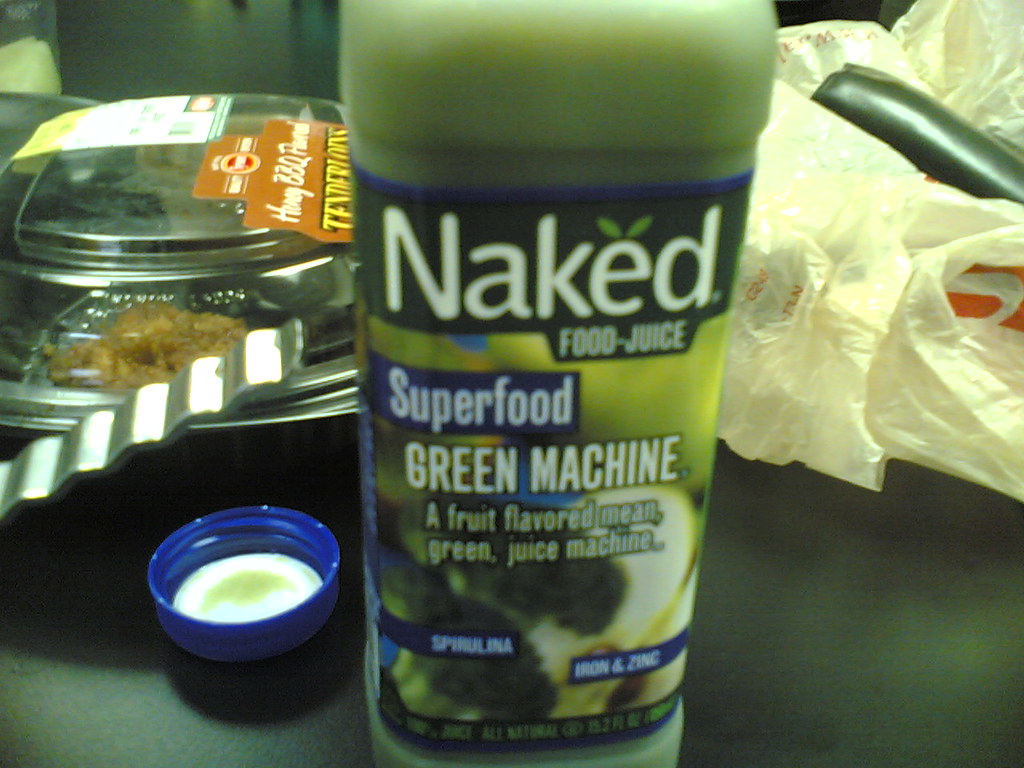An image depicting a bottle of Naked Juice, specifically the Superfood Green Machine variety, prominently displayed in the center. The bottle is missing its cap, which is placed nearby next to the container. The overall image quality is quite low. In the background, slightly out of focus, there's a package containing a single piece of fried chicken. To the right, a grocery bag with a black object perched on top is visible. A metal object protrudes into the frame from the left side of the photograph, positioned roughly in the middle. This cluttered and somewhat haphazard arrangement contrasts with the attempt to feature the juice bottle prominently.